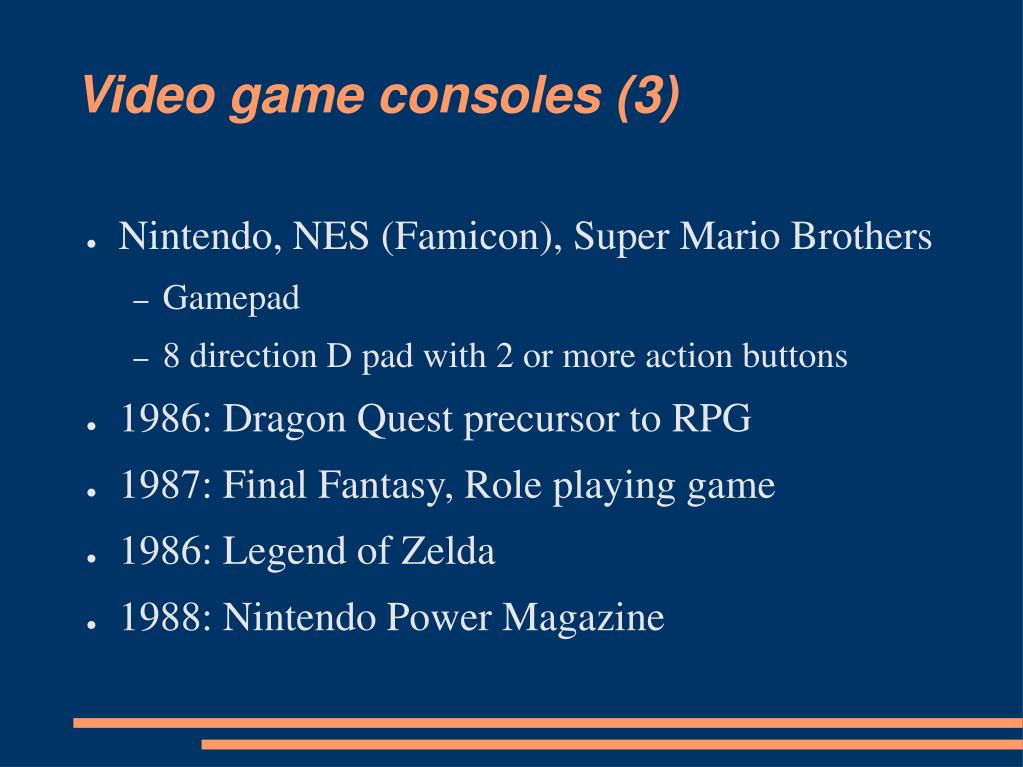The slide appears to be an independent slide from a PowerPoint presentation, designed with a dark blue background. The title "Video Game Consoles (3)" is prominently displayed at the top in pale orange, sans-serif italic font. Underneath, five bullet points in white serif font detail significant elements connected to video game consoles:

1. **Nintendo, NES (Famicom), Super Mario Brothers**
   - Gamepad
   - Eight-direction D-pad with two or more action buttons

2. **1986: Dragon Quest**
   - Precursor to RPG

3. **1987: Final Fantasy**
   - Role-playing game

4. **1986: The Legend of Zelda**

5. **1988: Nintendo Power Magazine**

At the bottom of the slide, two pale orange lines of differing lengths stretch across, echoing the color scheme of the title. This slide appears to catalogue key developments in video gaming history, albeit with a slightly disordered timeline.